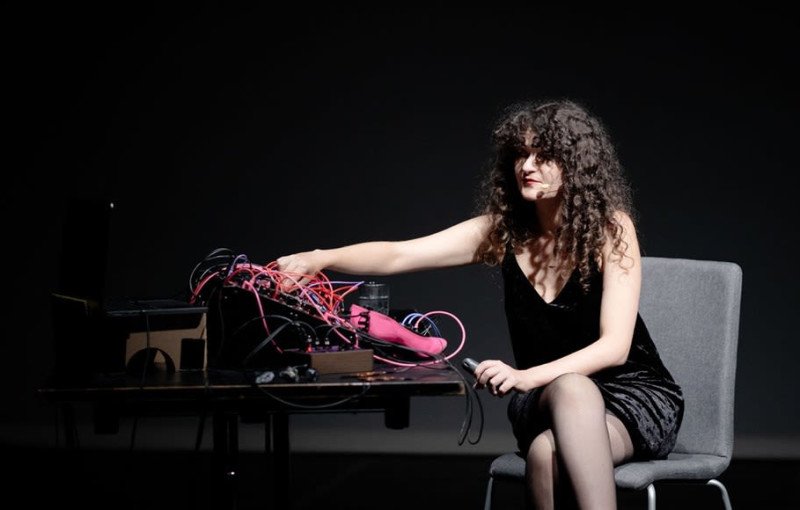In the image, a white woman with black curly hair sits angled left in a gray chair, wearing a black sleeveless dress. She holds a microphone in one hand, while her other arm reaches out toward a black contraption on a rectangular table beside her, entwined with various colored wires. Another microphone, attached via a thin rod with a white tip, is positioned near her mouth. Her legs are crossed, and her body faces the left. The background is entirely black, emphasizing the indoor setting of the shot. The colors in the scene include black, gray, pink, light blue, and brown.